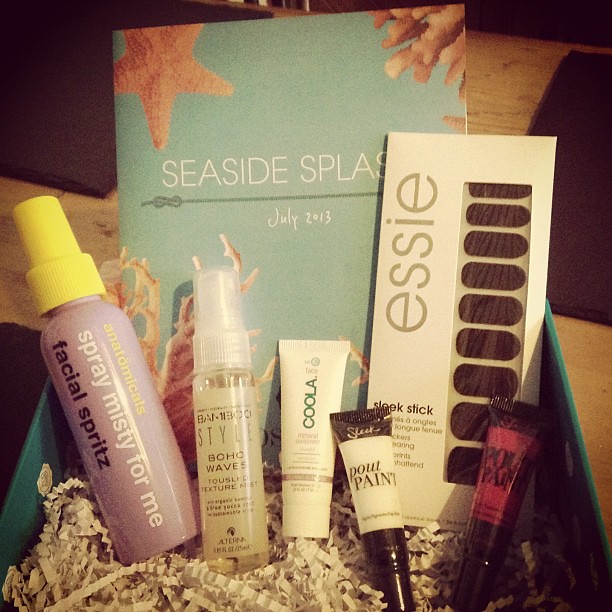This indoor photograph features a turquoise square gift basket resting on a wooden table adorned with dark brown placemats. The basket, approximately five inches high and four to five inches wide, is filled with shredded white paper for padding. Inside the basket is a neatly arranged selection of beauty products:

- A lavender-colored bottle with a yellow cap labeled "Anatomicals Spray Misty For Me Facial Spritz" in white and black font.
- A clear bottle with a cream-colored label that reads "Boho Waves Style."
- A small white tube with the word "Coola" branded vertically in green font.
- Two tubes of "Pout Paint": one white and black, and the other red and black.
- Behind these items, a white envelope with a see-through window displaying press-on nails, labeled "Essie" in gray font with the description "Sleek Stick" underneath.
- At the back of the basket, a light seafoam green, rectangular board featuring a starfish and coral images, with "Seaside Splash, July 2013" printed in the center in white lettering.

The composition of the basket and its contents is well-organized, making it an attractive gift set with a clear aquatic theme highlighted by the decorated board.